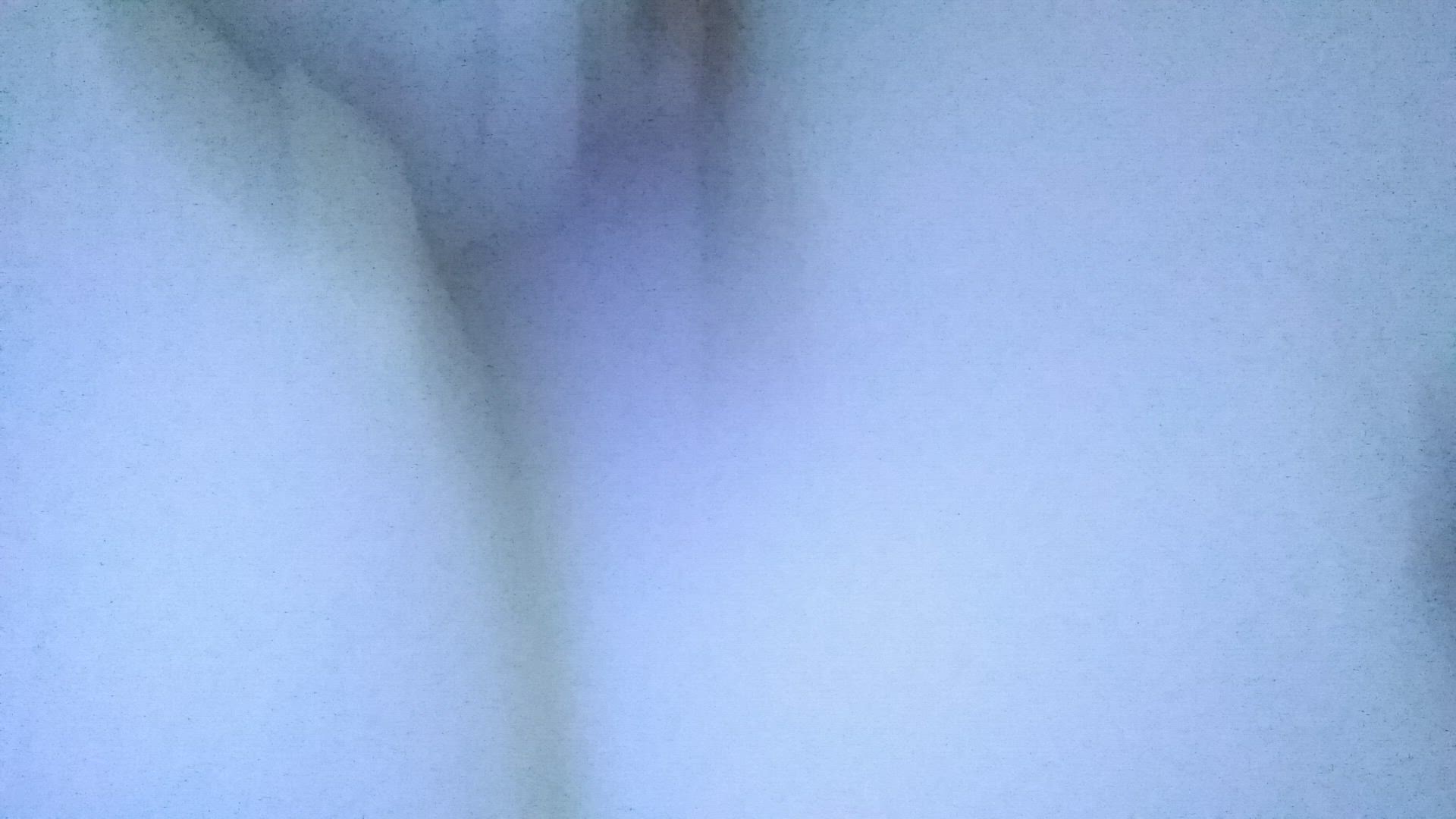This horizontal photograph features a soothing, light blue, hazy composition with an artistic touch. Dominating the left half of the image is a striking, Y-shaped haze punctuated by a darker blue vein, resembling the letter 'Y'. This vein exhibits textures that appear almost rocky or mineral-like, adding an element of natural intrigue. On the far right edge of the photo, subtle areas of slightly darker blue emerge, contributing to the image's mystique and complexity. Throughout the lighter blue areas, gentle, brighter spots subtly catch the eye, enhancing the overall calm and relaxing atmosphere of the photograph.